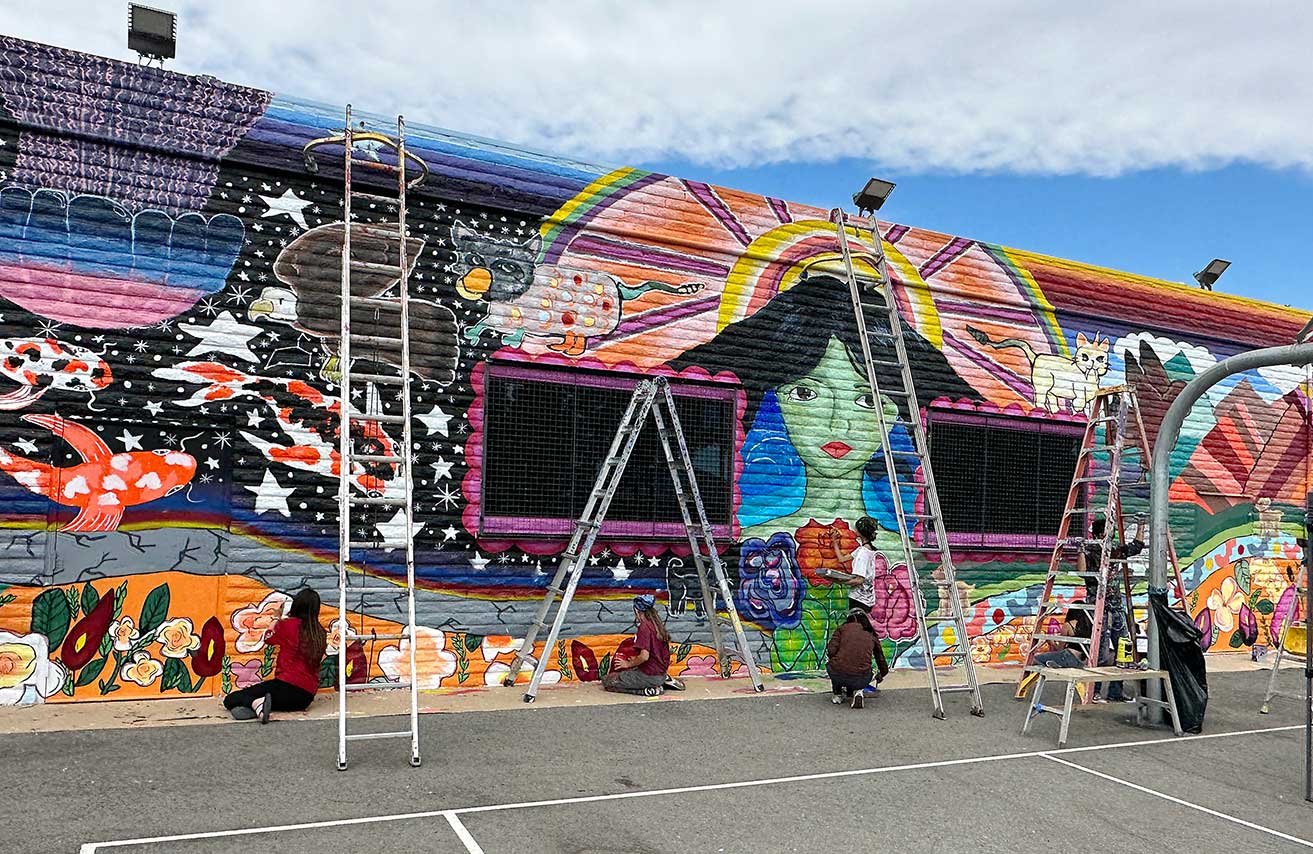In the photograph, we see a vibrant, large-scale mural being painted on the outside wall of a one-story brick building. The scene is set on a clear day with blue skies and some heavy clouds. Five artists, comprising three women and one man, are diligently working on different sections of the mural. The mural itself is a colorful and detailed street art composition spanning the entire side of the building. 

At the center of the mural stands an intriguing figure of a green-skinned woman with flowing dark black hair, illuminated by a bright sun directly above her. To her left, a goldfish or koi is depicted swimming against a black background dotted with white stars, creating an impression of an underwater scene. The lower part of the mural features serene flowers and a sandy walkway, adding an earthly element to the composition.

Multiple ladders are propped against the wall, allowing the artists to reach the topmost parts of the building. The combination of these diverse elements - the woman, the aquatic life, the floral and sandy motifs, all set against a backdrop of the day and night sky - results in a harmonious and captivating piece of public art.